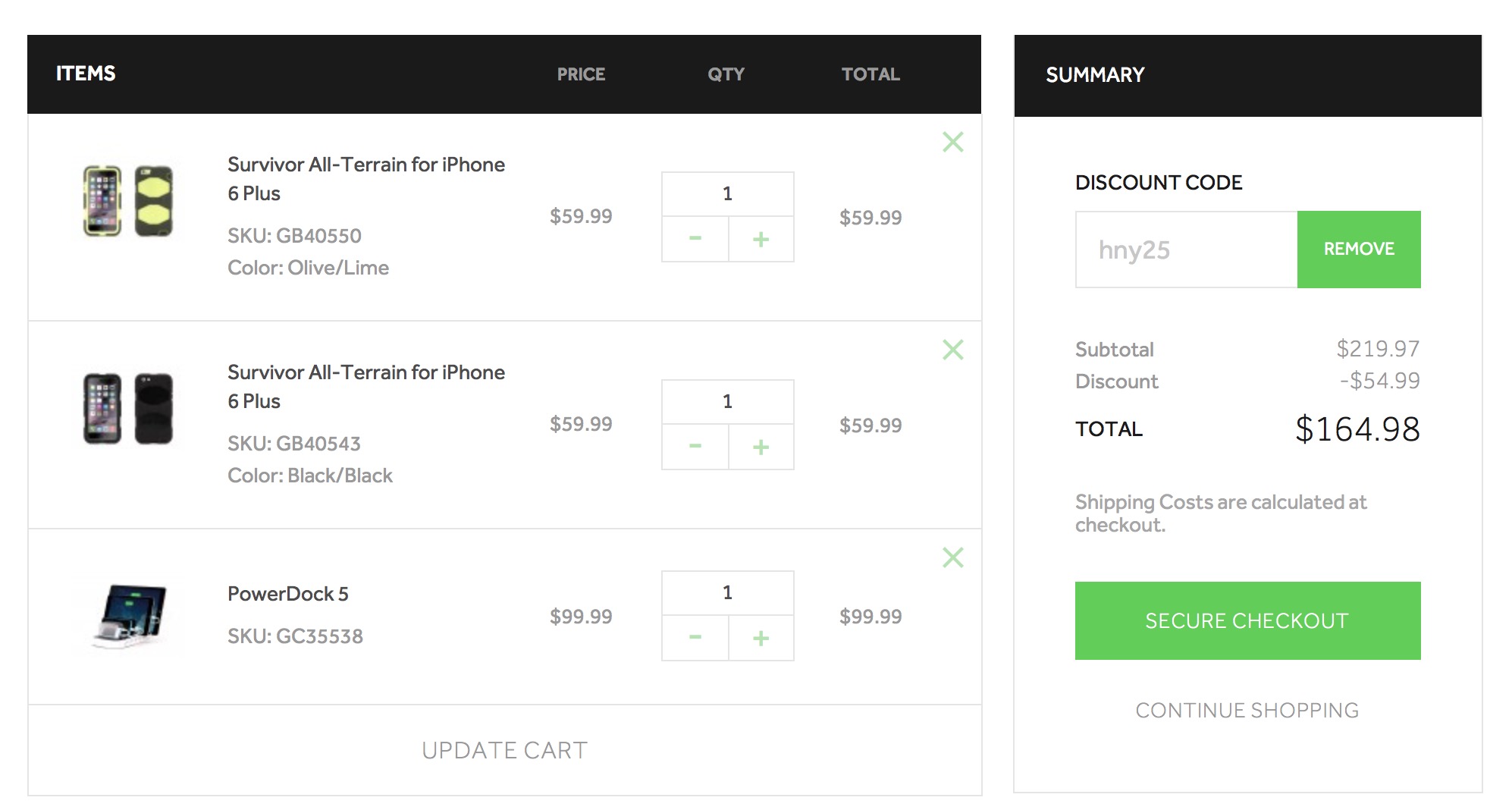**Order Summary Screenshot:**

The screenshot displays an order menu that lists three items along with their respective details, including price, quantity, and total cost.

1. **Item Details:**
   - **Product:** Survivor All-Terrain Case for iPhone 6 Plus
   - **SKU:** GB40550
   - **Color:** Olive Lime
   - **Price:** $59.99
   - **Quantity:** 1 
   - **Image Description:** The product image shows a durable, all-terrain case specifically designed for an iPhone 6 Plus.

2. **Item Details:**
   - **Product:** Another Survivor All-Terrain Case for iPhone 6 Plus
   - **SKU:** Not specified
   - **Color:** Olive Lime
   - **Price:** $59.99
   - **Quantity:** 1 
   - **Image Description:** Similar durable, all-terrain case for an iPhone 6 Plus.

3. **Item Details:**
   - **Product:** Power Dock 5
   - **Price:** $99.99
   - **Quantity:** 1
   - **Image Description:** A charging dock capable of charging five devices simultaneously.

**Pricing Summary:**
- **Subtotal:** $219.97
- **Discount Code:** HN25 applied which gives a discount of $54.99
- **Discounted Total:** $164.98
- **Note:** Shipping costs are calculated at checkout.

**Interactive Options:**
- **Secure Checkout:** A green button likely intended to proceed with payment.
- **Continue Shopping:** An option to add more items to the order.

This detailed caption provides a comprehensive understanding of the screenshot, describing each item, prices, discounts, and interactive buttons available.